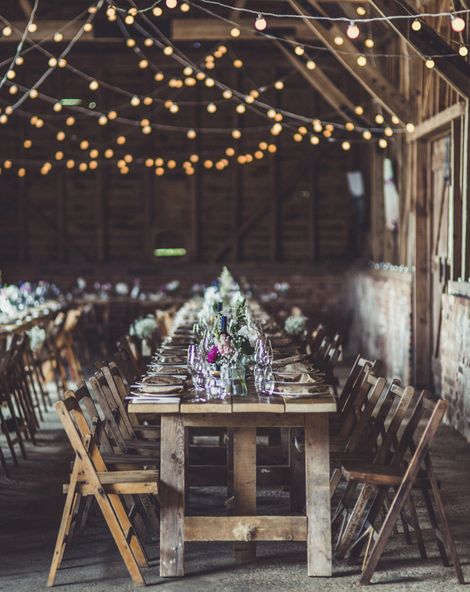The vertically aligned rectangular image depicts an indoor setting designed for a celebration, possibly a wedding, reminiscent of a rustic barn or large, stone-floored room. The ground appears to be concrete, and the space features long, brown wooden tables with matching wooden chairs, all bearing signs of age and wear. These tables, arranged in various orientations, are adorned with detailed place settings that include plates, napkins, and floral centerpieces comprising purple and white flowers. The middle of the photo prominently displays a banquet table set for a large gathering, stretching from the foreground to the background. Another table is partially visible to the left, slightly out of focus, while a third table stands perpendicularly against the far wall. Above the tables, strings of round, yellow-orange lights with white wires are draped across the ceiling, casting a warm glow over the scene. The lower portion of the walls is constructed from brown stone, adding to the rustic ambiance, while the upper sections are made from wooden planks akin to those in a wood cabin. There are no people seated or food served, further emphasizing the anticipation of the impending celebration.